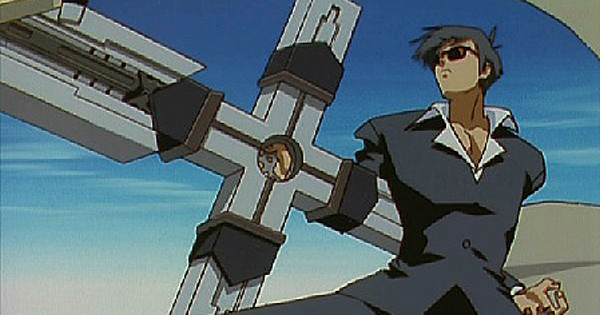The screenshot appears to be from an anime and depicts a character situated on the right-hand side of the frame. The image is of notably low quality, featuring jagged lines and poor resolution. The character is a man with light Caucasian skin, clad in a black suit coat that is unbuttoned at the top, revealing a partially open white collared shirt beneath. His attire includes black pants and black sunglasses, complementing his short but spiky gray hair. He is grasping a large silver cross in his left hand. The cross is crafted from silver metal and features intricate etching lines along its length. Near the center of the cross, there are black brackets from which lines extend towards a recessed hole located at the very center. The man's appearance and the massive silver cross, which could be mistaken for a large weapon or staff, draw significant attention in this scene, accentuating his formidable presence.